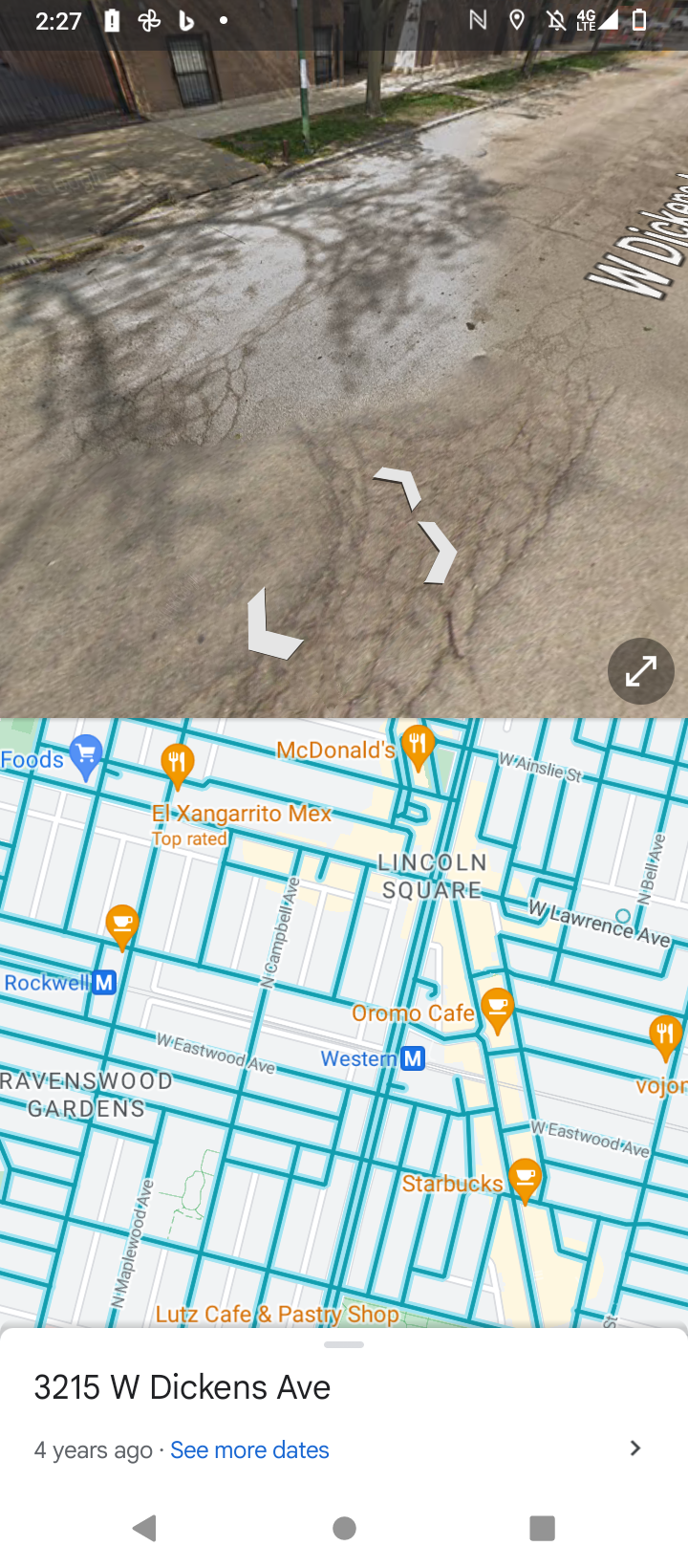This is a detailed screenshot of a mobile device displaying both a street view and a drawn map of an urban area. The top portion of the screenshot features the street view, showcasing W. Dickens Road with visible residential housing or apartments on the left side. The road appears worn and has visible cracks. The device's notification bar indicates a low battery, with the time stamped at 2:27. The user has their location services enabled, notifications turned off, and the device is connected to a 4G LTE network. Additionally, the photo gallery app is open.

In the bottom section of the screenshot, the map features blue outlines highlighting key locations such as Lincoln Square, McDonald's, Ravenswood Gardens, and Luke's Cafe and Pastry Shop. The map section provides a drawn representation of the streets and points of interest correlating to the street view above.